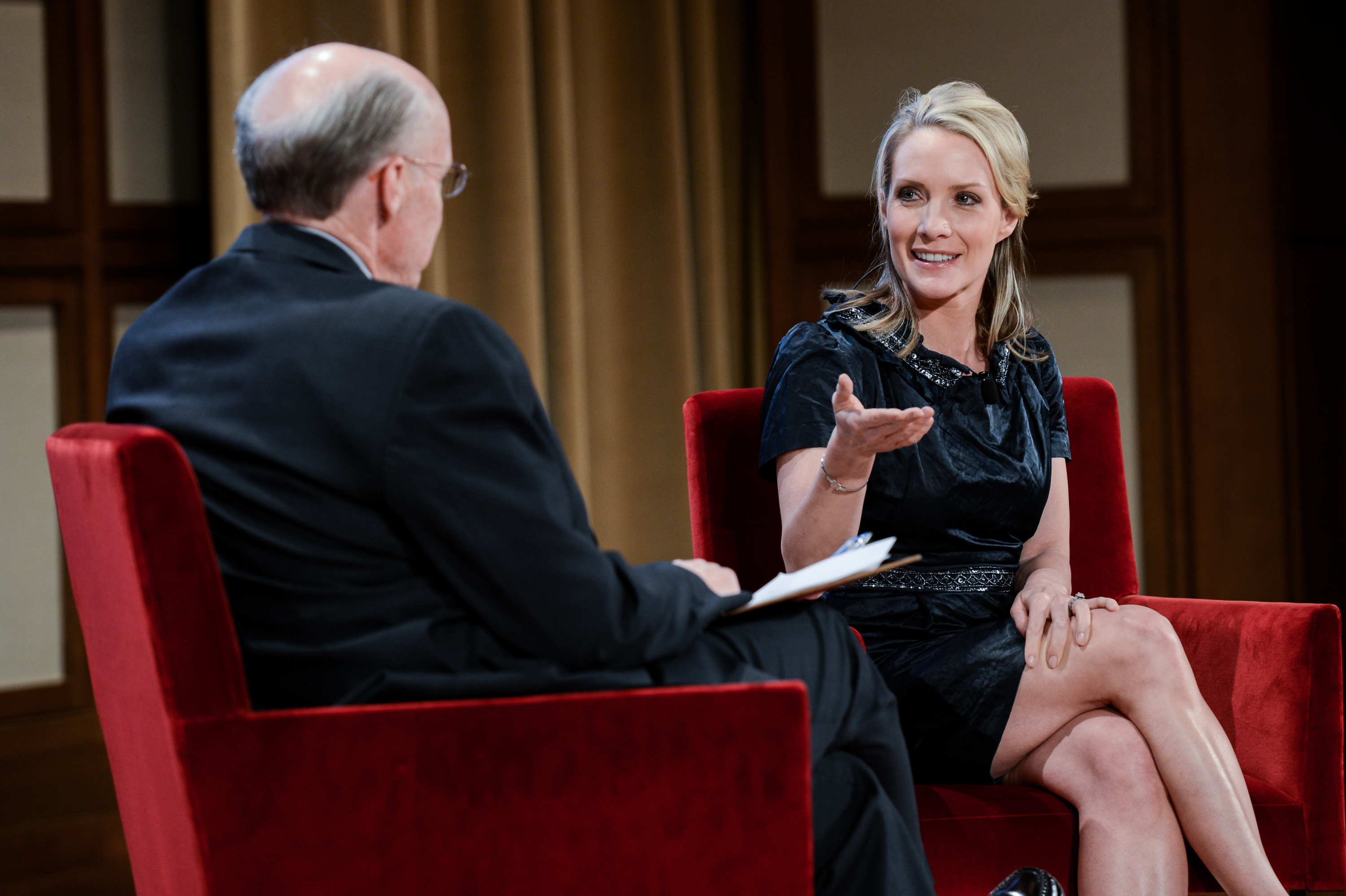In the photograph, two people are seated in a talk show-like professional setting, both on high-backed red velvet chairs. The man, positioned on the left, is facing the woman on the right. He is balding with a shiny crown, wears glasses, and is dressed in a dark blue or black tuxedo, dark blue dress pants, and black dress shoes. His right arm rests on a piece of paper on his lap, and his right leg is crossed over his left. The woman on the right appears to be Megyn Kelly, with her blonde hair pulled back, dark brown eyes accentuated with eyeliner, and wearing a black dress with a belt. She sits with her right knee crossed over her left and a bracelet on her right arm. Her right hand is extended with the palm up, gesturing as she speaks, while her left hand rests on her knee. The background features long yellow curtains hanging over what seems to be a white and brown wooden wall, suggesting a studio environment. Both individuals are engaged in an active conversation.